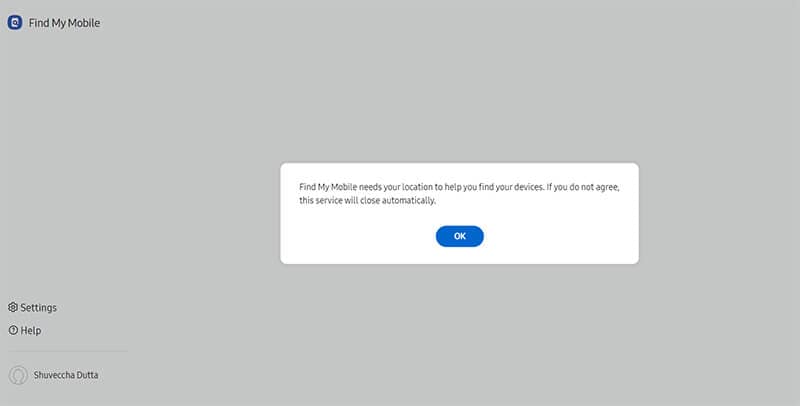Screenshot from the Find My Mobile App: 

The image is a screenshot taken from the Find My Mobile app, likely on a desktop or tablet. The main portion of the screen is darkened, indicating the areas that are currently not interactive. Centered prominently in the middle of the screen is a white, rounded rectangular pop-up dialog box.

The dialog box contains a message stating: "Find My Mobile needs your location to help you find your devices. If you do not agree, the service will close automatically." Below this message, there is a blue, rounded button labeled "OK" prompting the user to click it to proceed.

In the non-interactive, darkened background, additional interface elements are visible. On the left-hand side, there are icons for "Settings" and "Help," with the "Settings" icon at the top and the "Help" icon, represented by a small question mark inside a circle, just below it. At the very bottom left-hand corner, the profile name "SHUVECHA DUTTA" is displayed.

The clear demarcation between the highlighted pop-up and the deactivated background, along with the coherent visual arrangement, emphasizes the user prompt while providing context through the visible but inactive interface elements.